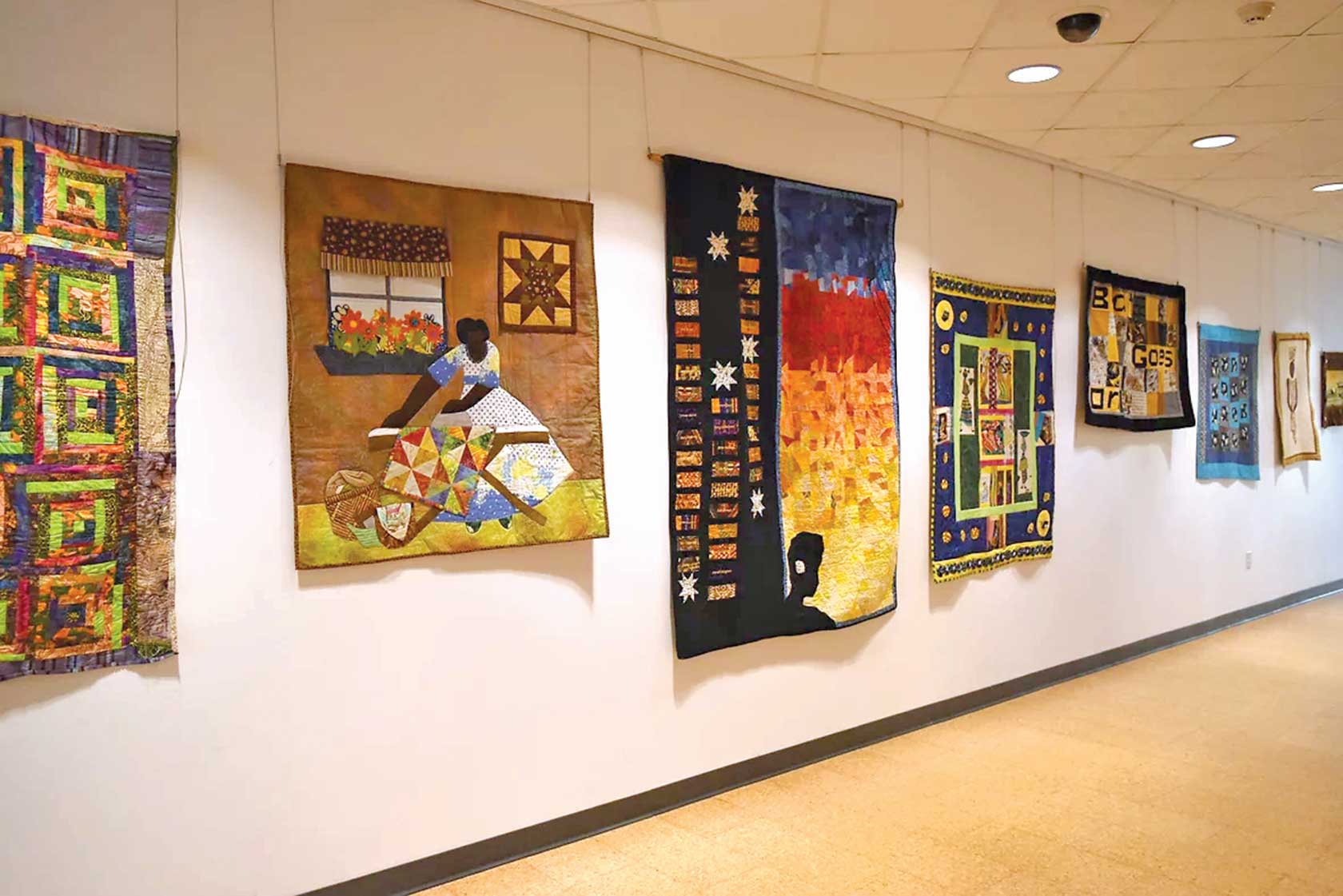This photograph captures an exhibit at an art museum, showcasing a series of quilts hanging on a solid white wall, which features a thin brown border at the bottom. The floor is made up of bright wooden planks. There are eight quilts visible, each intricately detailed, blending traditional and narrative styles. 

On the far left is a quilt with a classic log cabin pattern. Adjacent to it is a quilt depicting a woman sitting outside a house adorned with flowers on the windowsill, engaged in quilting. Another nearby quilt transitions from blue to red to orange to yellow, illustrating either a silhouette of a person or a tree. Additionally, there's a quilt featuring a blue square with a green center and another with blue squares and flowers. One quilt shows a woman in a brown room wearing a white dress, while another features a bold pattern resembling a person's head leaning forward. There is also a piece with some indecipherable lettering. 

Overall, the exhibit seems to explore the versatility of quilt art, blending traditional patterns with intricate scenic and abstract designs.